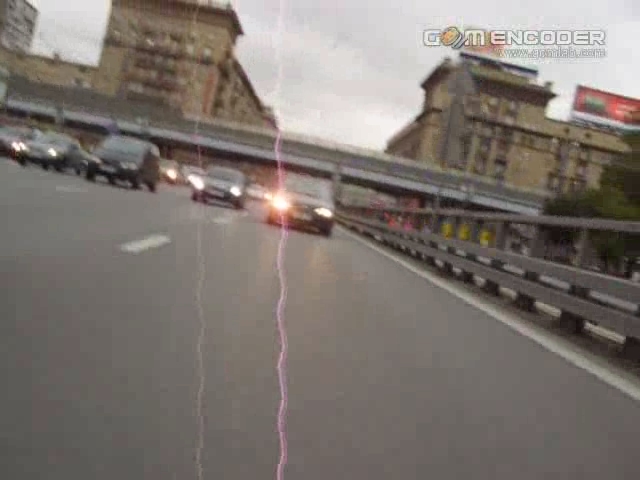This photograph captures a bustling, four-lane highway during the twilight hours, with vehicles traveling towards the camera, their headlights glowing in the fading light. The road is flanked by beige buildings on either side, several stories tall, and features prominent billboards, including a red and white one atop a building on the right. Overhead, a crosswalk or bridge spans the highway, creating a visual bridge in the composition. A guardrail runs along the right side of the road, with a dotted white line marking the lanes on the left. A faint and bold pink line, resembling a lightning strike, runs vertically down the center of the image, adding a surreal touch to the cityscape. The setting appears to be somewhere in the UK, as suggested by the front license plates on the cars. A banner at the top of the image reads "Gem Encoder," accompanied by a blurry URL. Above, the sky is a mix of bluish-gray clouds, hinting at the approaching night.